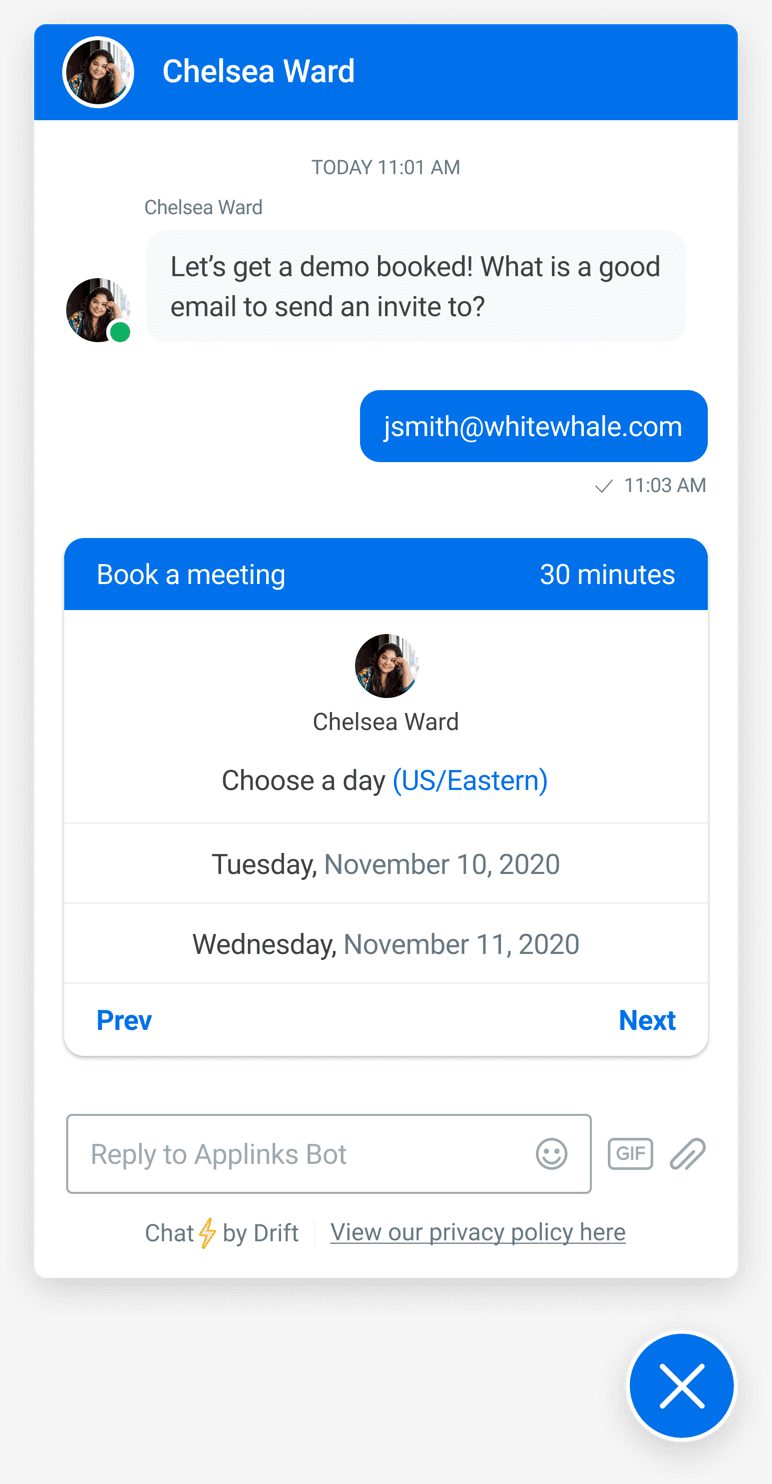The image depicts an instant messaging screen where a user receives messages from Chelsea Ward. Chelsea’s profile picture features a circular portrait of a dark-haired woman with a light skin tone, wearing a colorful blouse. At 11:00 AM, Chelsea suggests scheduling a demo and asks for a good email to send the invite. The user replies with "jsmith@whitewhale.com" at 11:03 AM. 

Chelsea then provides options for a 30-minute meeting on either Tuesday, November 10th, 2020, or Wednesday, November 11th, 2020, specifying that the times are in US Eastern Time. They are using the AppLinks bot, which has options to send an emoji, a GIF, or an attachment, and it mentions features like "chat by GIF" and a link to view the privacy policy.